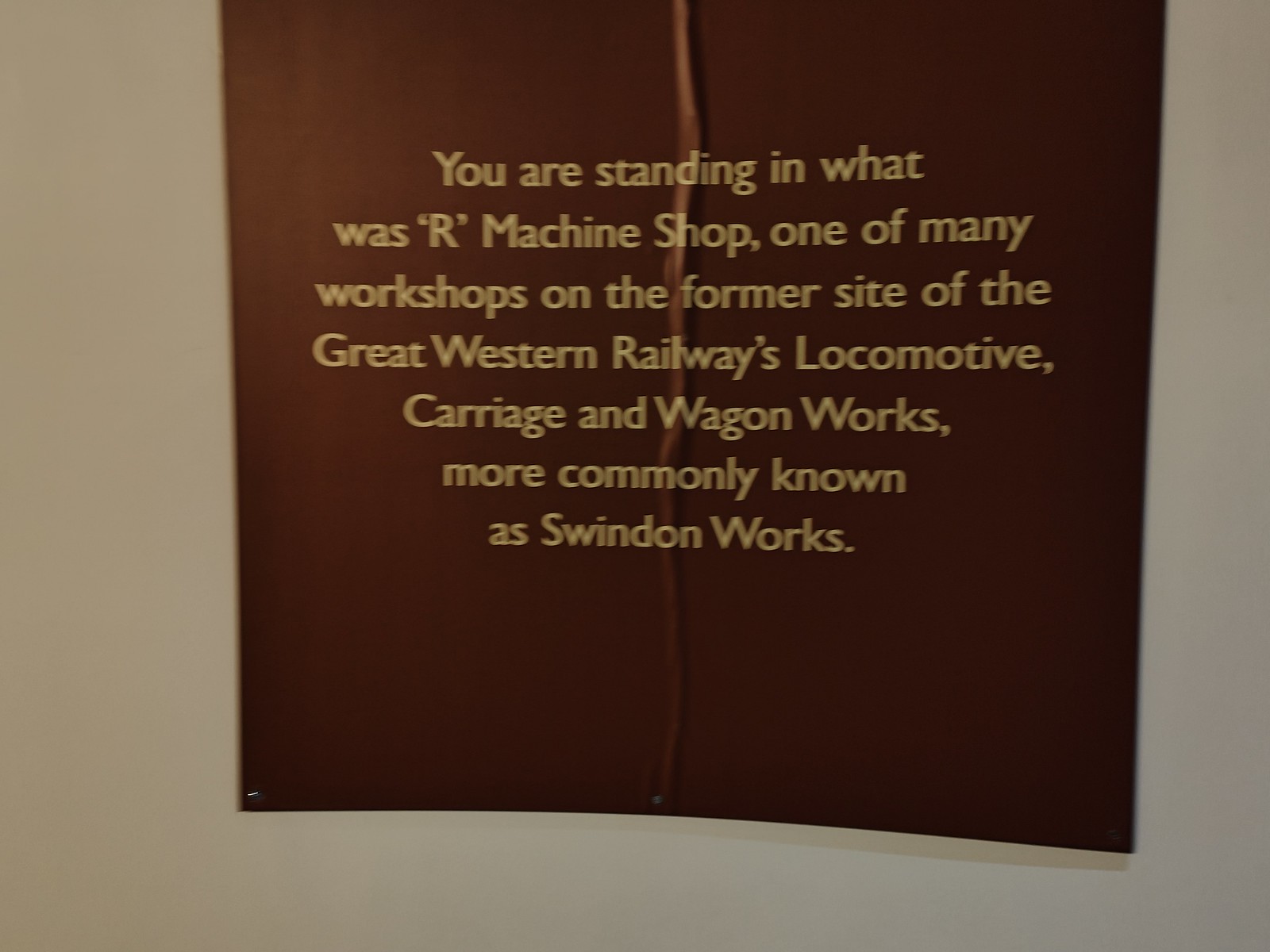The image depicts a maroon-red square sign mounted on an off-white, cream-colored wall, likely within a historical building or museum. The sign appears to have a crease running vertically through its center, possibly due to a missing nail on the left side. The sign's gold lettering reads: "You are standing in what was our Machine Shop, one of many workshops on the former site of the Great Western Railway's locomotive, carriage and wagon works, more commonly known as Swindon Works," with the letter 'R' in "Machine Shop" enclosed in parentheses.